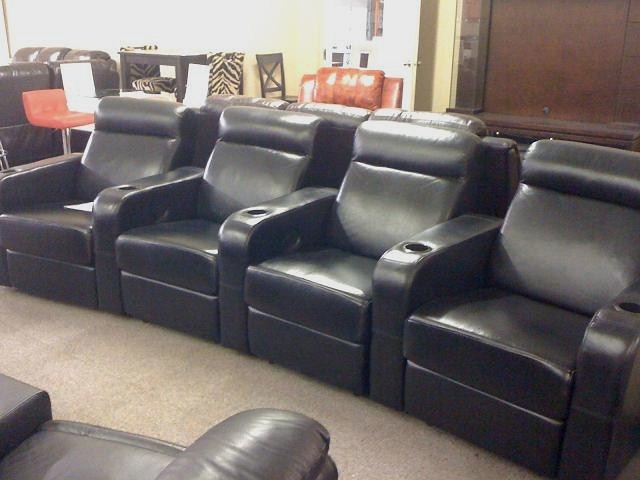The image depicts the interior of a furniture showroom, prominently featuring a set of four black leather reclining theater chairs arranged in a slight curve. These luxurious chairs are designed with cup holders in their arms, including extra holders between the connected seats, for a total of five cup holders. They are heavily cushioned, providing comfort similar to that of cinema seating. Beneath the chairs is a light brown carpet, and in the distant background, various other furniture pieces are visible, including dining chairs with zebra-print backs, a red leather bar chair, and a brown leather sofa. A partially open door in the background reveals a room containing white appliances. The right side of the picture is dominated by a brown wooden wall, which may be a display case.